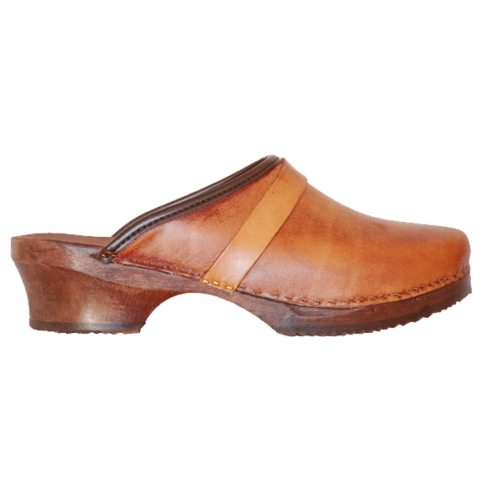The image features a single brown leather clog positioned centrally against a white background. The clog, which shows the front of the shoe facing to the right and the heel to the left, is designed as a slip-on with an open back, resembling a slipper with no strap to hold the heel. It showcases a wooden sole and a thick hard rubber bottom. The brown leather upper includes a decorative strap for added detail. Visible stitching runs along the side, highlighting the craftsmanship. This detailed presentation, devoid of any text, suggests that the shoe could be a woman's design and resembles the kind typically seen on clothing retail websites.